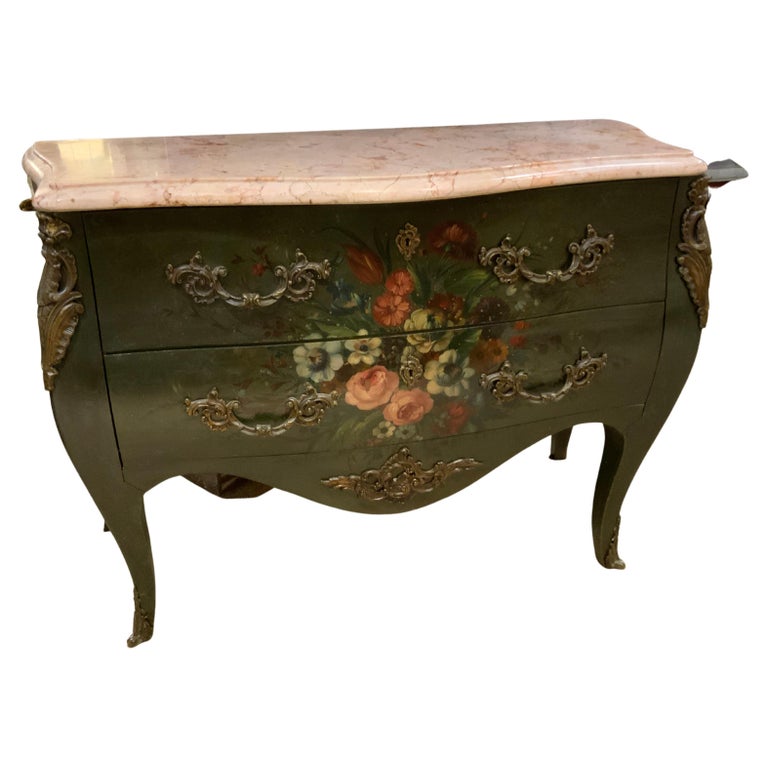The image depicts an ornate, antique chest of drawers set against a solid white background. It features a dark green or dark cherry wooden frame with a curved, elegant design. The chest stands on four slightly curved legs, each adorned with brass hardware that matches a decorative metal piece on the chest's bottom. 

The chest has two drawers, each fitted with two vertical, ornate brass handles and a matching brass keyhole escutcheon. Between the two sets of handles, a lavishly painted bouquet of flowers, including pink roses, white daisies, orange, blue, yellow, red, and deep purple flowers, is prominently displayed in a 17th-century style. 

The entire piece is topped with a beautifully veined marble surface in a pinky-white or light brown shade, complementing the intricate floral and brass accents. This chest of drawers, with its antique finish and detailed craftsmanship, presents a harmonious blend of florals and refined elegance.